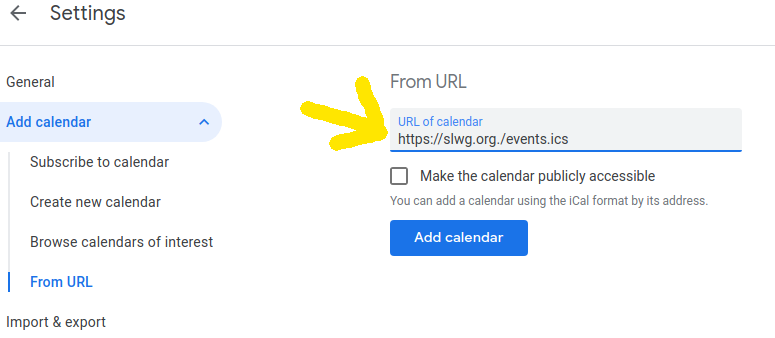The image features a minimalist interface with a white background. At the top left corner, a sentence is displayed, accompanied by an arrow pointing to the left. A thin gray line stretches horizontally from the left to the right. Below this line on the left side, the word "General" is written, followed by a blue section with the phrase "Add Calendar" written in darker blue text. Underneath this, in black text, are the options "Subscribe to Calendar," "Create New Calendar," and "Browse Calendars of Interest." Below these options, there is a blue text link that says "From URL." Beneath this, "Import and Export" is written in black text.

On the right side of the image, "From URL" is written again, followed by a light gray input box highlighted with a blue line at the bottom. Inside this box, in blue text, it says "URL of calendar." Below the input box, in black text, it displays an example URL: "https://slwg.org/events.ics."